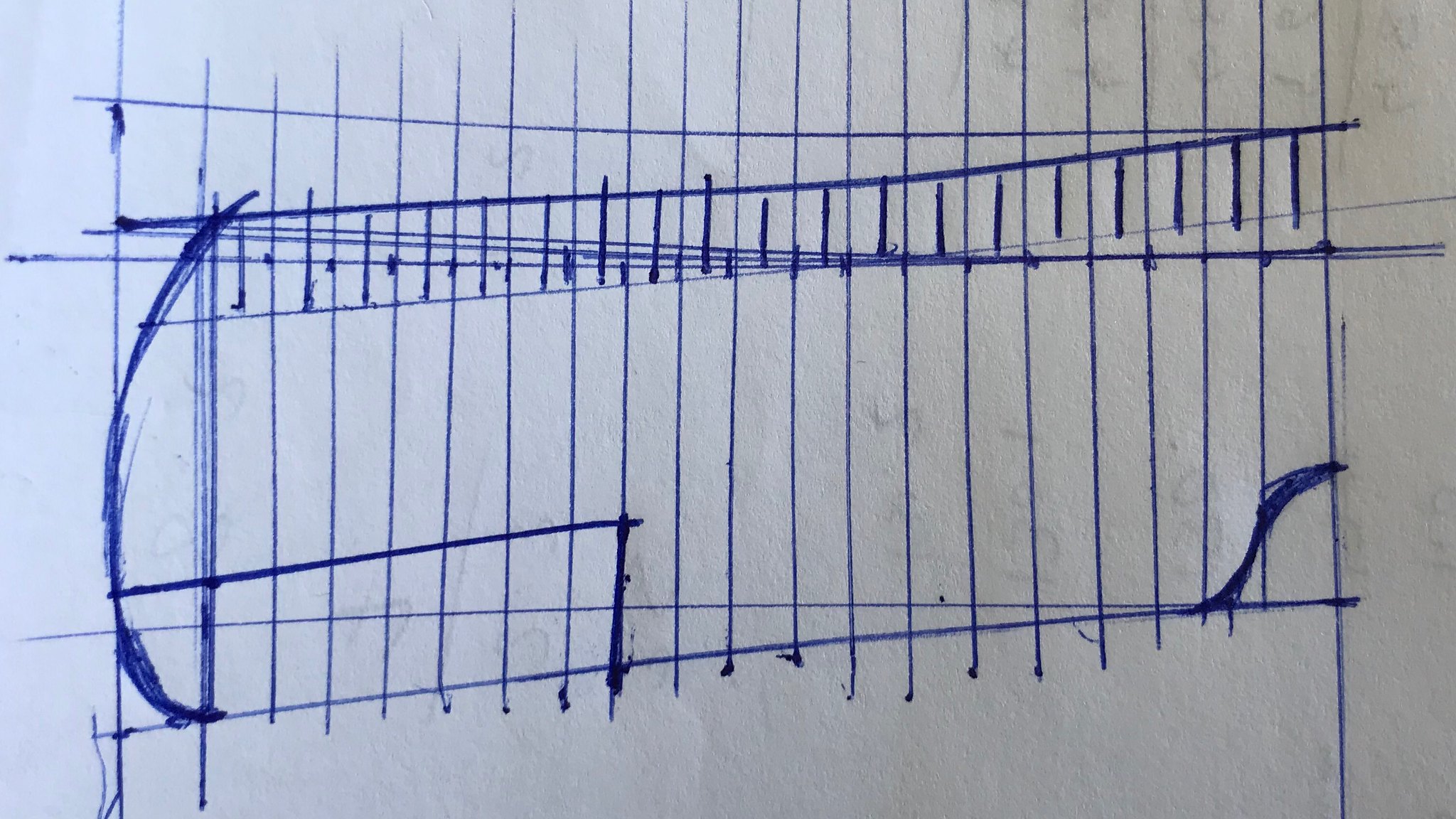The image features a meticulously drawn design on a plain white sheet of paper using blue ink. Central to the composition are multiple long vertical lines that stretch almost the entire height of the page, running parallel to one another. Near the top, a thin horizontal line intersects these vertical lines, while slightly below it, a darker horizontal line extends at an upward angle, creating a triangular shape at the right edge where the two lines meet.

From this second horizontal line, several dark blue vertical lines dangle downward in a manner reminiscent of hanging threads. On the left side of the paper, there is a partial arc, suggesting a segment of a circle, although it does not form a complete semicircle. Towards the bottom left corner of the page, a small rectangular shape is formed by one horizontal and one vertical line.

On the right side, beneath the vertical lines, a dark, curvaceous line swirls from the bottom of the vertical lines, extending and curling towards one of the vertical strokes. The overall design consists of various blue lines, both straight and curved, creating an abstract and intricate pattern against the stark white background of the paper.